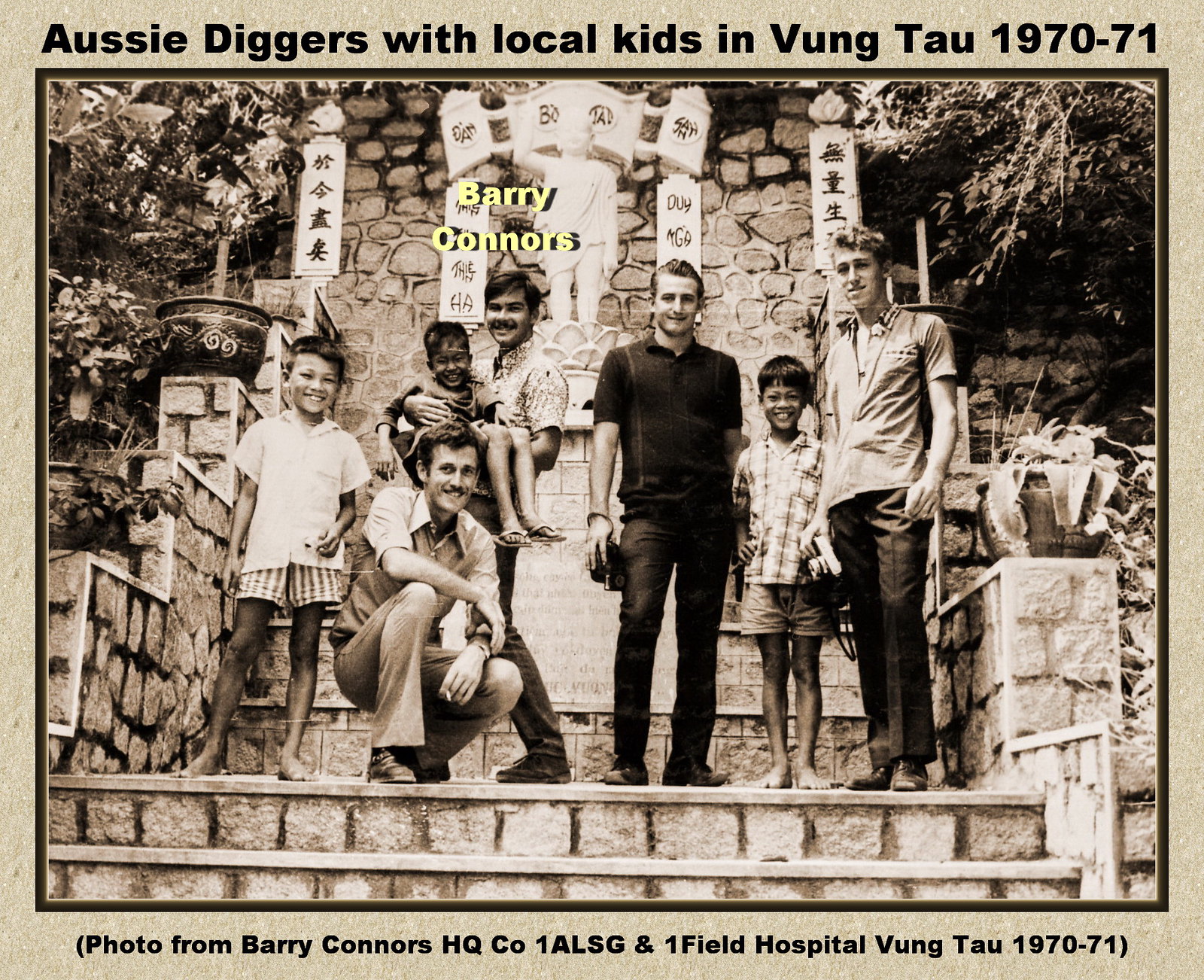The image depicts a postcard-sized, beige card featuring a black-and-white photograph with a gray border. The photo’s caption at the top reads: "Aussie Diggers with local kids in Vung Tau, 1970-71," and at the bottom, it states: "(Photo from Barry Connors HQ CO 1ALSG and 1 Field Hospital Vung Tau, 1970-71)." The scene portrays four adults and three children outdoors in Vung Tau, Southeast Asia. In the background, a stone staircase leads up a steep hillside adorned with oriental symbols on vertical boards, pots, and a statue amidst rocks, grass, and trees with creeping vines. One adult is holding a child, while another, with a mustache, is seen squatting with a cigarette. The adults and children, two of whom are wearing collared shirts and shorts, all smile warmly at the camera, conveying a moment of camaraderie.